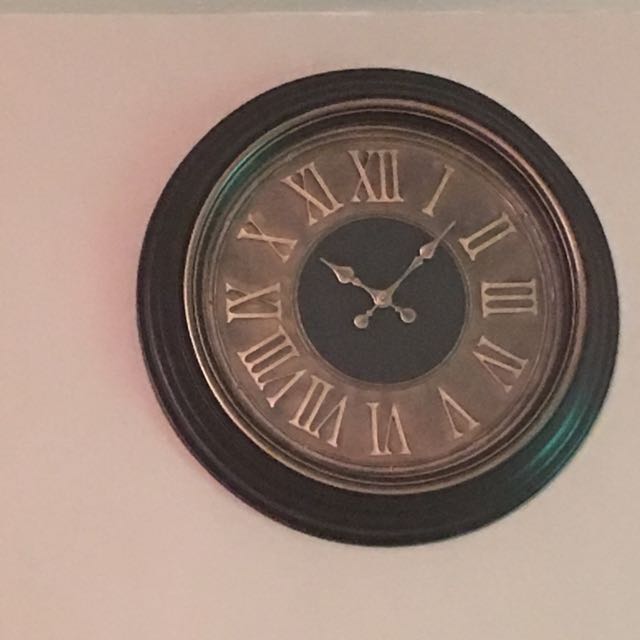The image showcases a clock adorned with gold-colored Roman numerals and hands. The clock's design features a dark brown frame and an interior ring with a rusty gold tone, contrasting beautifully with its almost jet-black center. It's positioned against a slightly beige wall. The shorter hand points towards X (10) and the longer hand rests between I and II (1 and 2), making the time approximately 10:07. The clock stands out on the right side of the image, suggesting a homely or workplace setting.